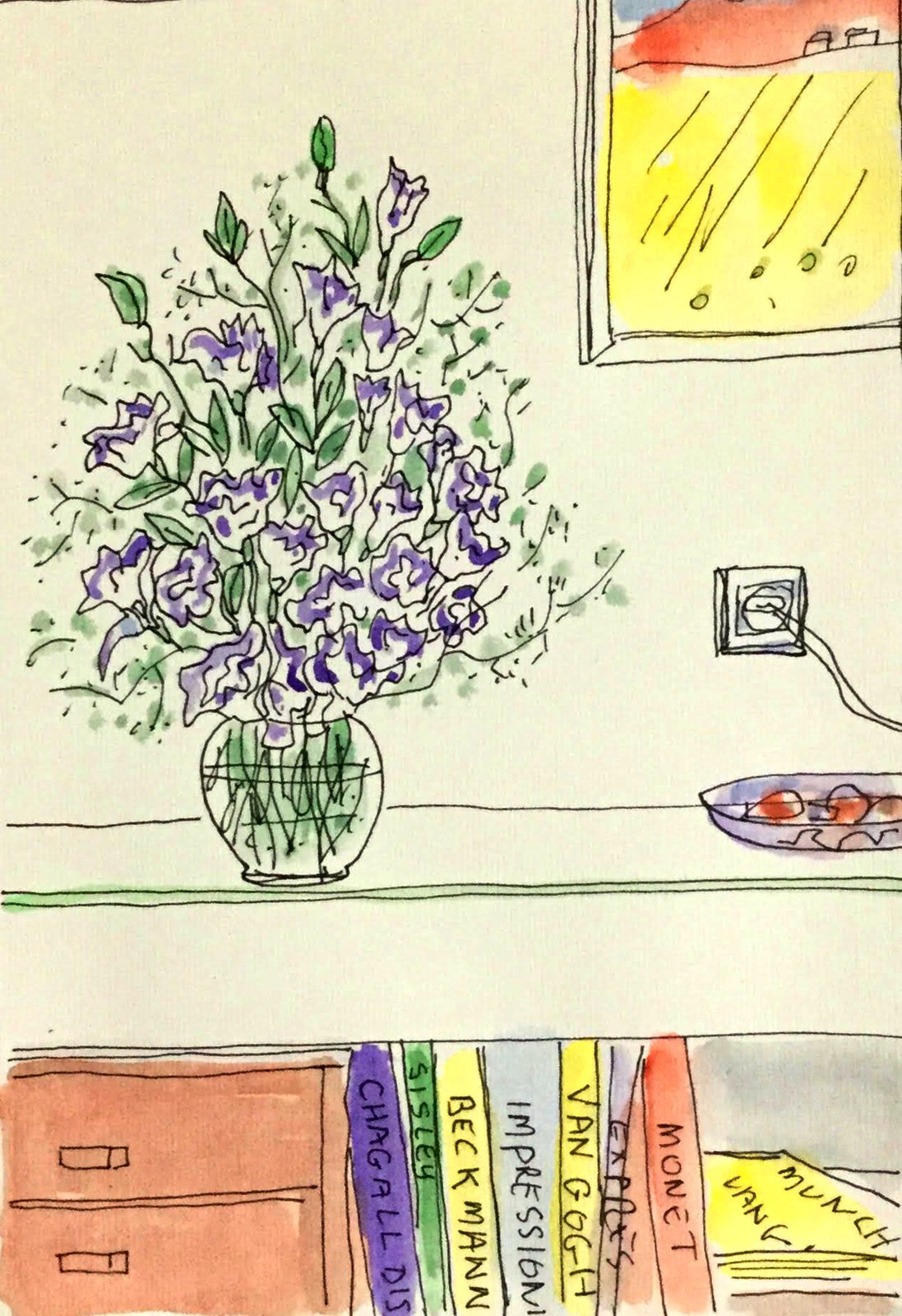The large rectangular watercolor painting depicts a still life scene in a living space, showcasing a clear, bulbous vase filled with purple flowers and green leaves. The flower tips are shaded in purple, and the leaves and stems are outlined in black with the green hue visible through the clear water in the vase. The vase rests on a shelf, also outlined in black, with a plug socket visible on the right. A small purple bowl containing reddish berries or fruits is positioned to the far right on the shelf. 

In the upper right corner, a framed painting with a yellow field, a red hill, and black lines suggesting crops hangs on the white wall. Below the main shelf, a secondary shelf holds two brown drawers and several vertically placed books leaning against them, with one book lying horizontally. The book titles include notable names like Monet, Van Gogh, Impressionism, Beckmann, and Sisley, adding an intellectual touch to the setting. The entire scene is delicately rendered with black outlines and watercolors, highlighting the tranquil and artistic atmosphere of the room.